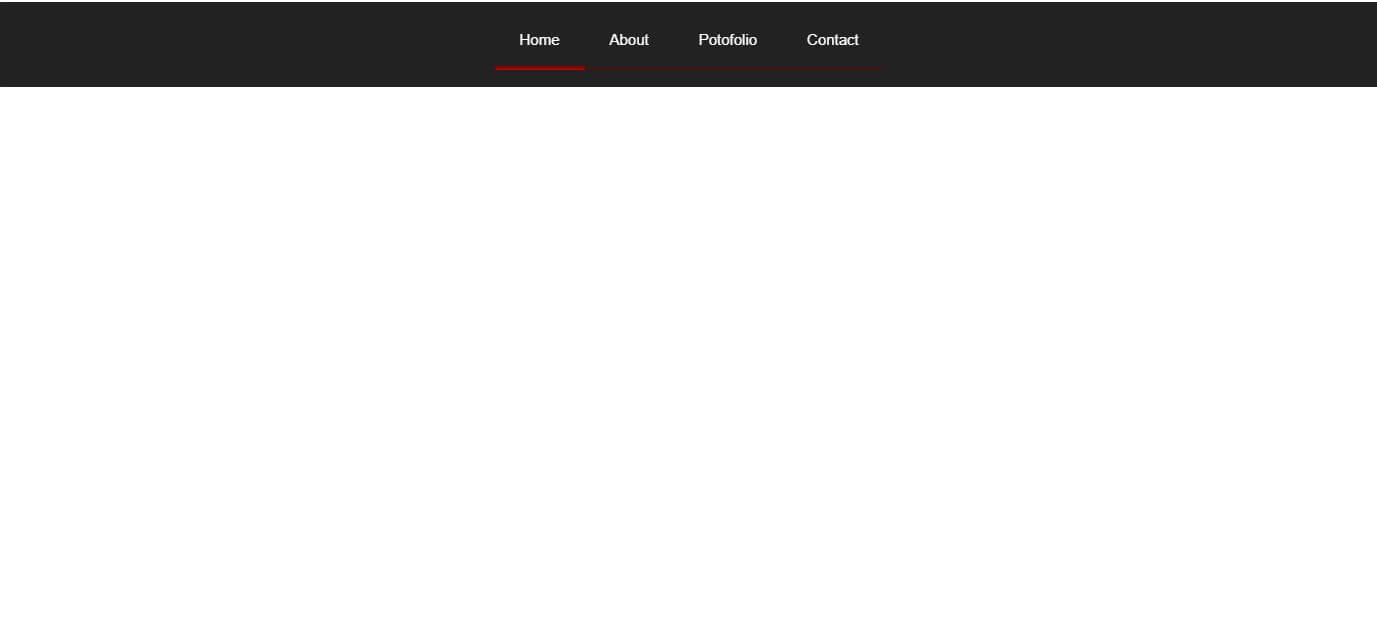The image depicts a minimalist webpage with a predominantly white background. A black bar, approximately one inch in height, spans the top edge of the page. This black bar contains four navigation links: "Home," "About," "Portfolio," and "Contact." The "Home" link is distinguished by a bright red underline, indicating the active page. The other links - "About," "Portfolio," and "Contact" - also feature red underlines, but they are darker and less prominent, suggesting they are not currently selected.